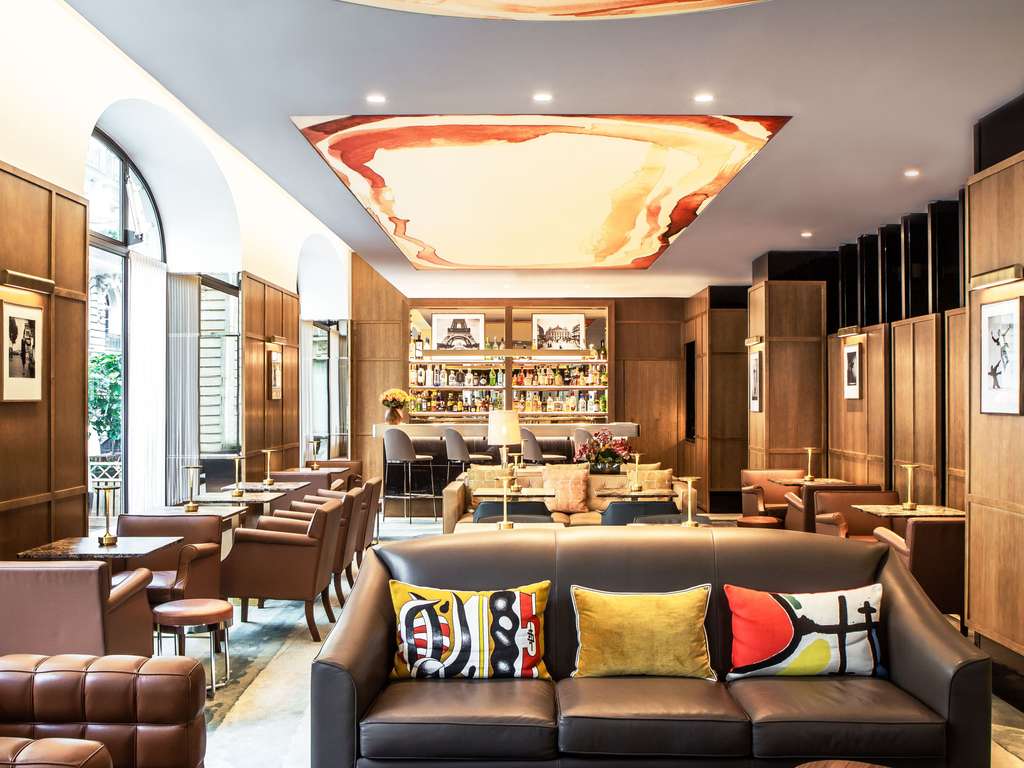The image showcases a striking stone-built structure, likely a historic apartment building or hotel, situated at a street corner. The building's exterior features a distinctive blend of light gray, beige, and pinkish hues, with its facade crafted from large tan bricks. The corner, prominent in the shot, gracefully curves around in a semicircle, and extends upwards to at least six stories. Each floor is adorned with numerous balconies, fronted by elegant black wrought iron railings, and accessed through French doors or large glass doorways. The roof is primarily flat, but the corner culminates in a domed roof section, suggesting a penthouse suite, adding a crowning touch to the structure. The photograph, taken during a brilliantly sunny day with a clear blue sky, highlights the building's grandeur from street level up to its impressive roofline.